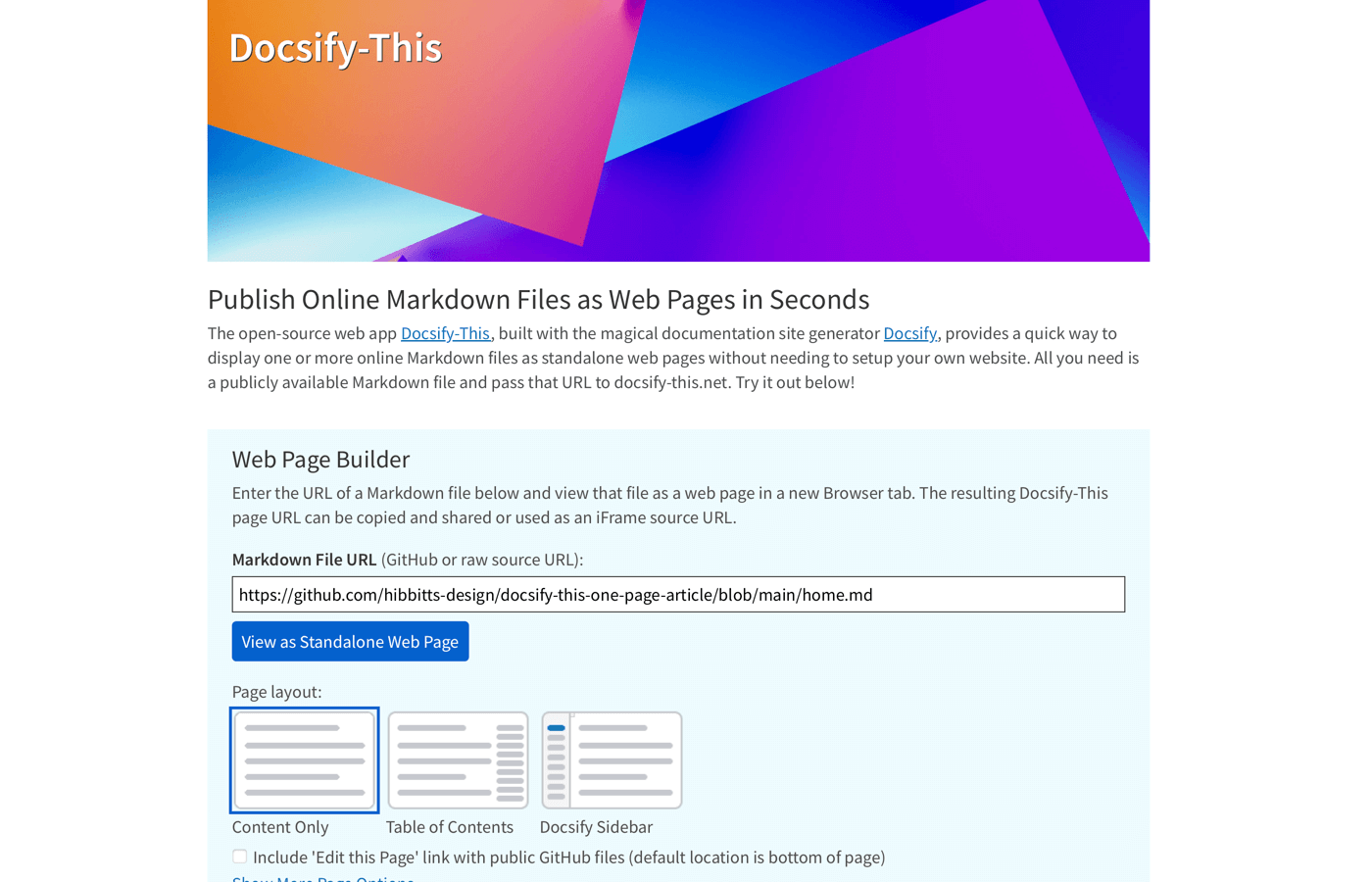**Image Caption:**

At the top, there's a vibrant rectangle displaying a mix of colors including orange, purple, blue, light blue, and white, along with some abstract shapes. The text within this rectangle reads "Docsify - This." Below this colorful banner, a tagline states, "Publish online markdown files as webpages in seconds."

Underneath the tagline, there's a paragraph with content that is mostly illegible due to the small font size, but some parts are highlighted with blue, underlined text while the rest remains in black. Proceeding further down is a blue rectangle labeled "Webpage Builder." Instructions within this section prompt users to enter the URL of a markdown file to view it as a webpage in a new browser tab. It suggests that the resulting Docsify page URL can be copied, shared, or used as a frame source URL. Specifically, it mentions "Markdown File URL" in parentheses, indicating it can be a GitHub or raw source URL.

Adjacent to this section, there's a dark gray-outlined rectangle resembling a website interface. Below it, another blue rectangle states "View as Standard Webpage." Under this, "Page Layout" is displayed with a visual representation composed of blue and gray lines, labeled "Content Only."

Further down, there's a white rectangle with gray lines inside, titled "Table of Contents." Next to this, a combination of a gray and a white rectangle is seen. The gray rectangle contains several dashes, with the first dash highlighted in blue and the rest in gray. The white rectangle beside it features gray lines and is labeled "Docsify Sidebar."

Lastly, there's a white square that reads, "Include 'Edit this page' link with public GitHub files. Default location is bottom of the page."